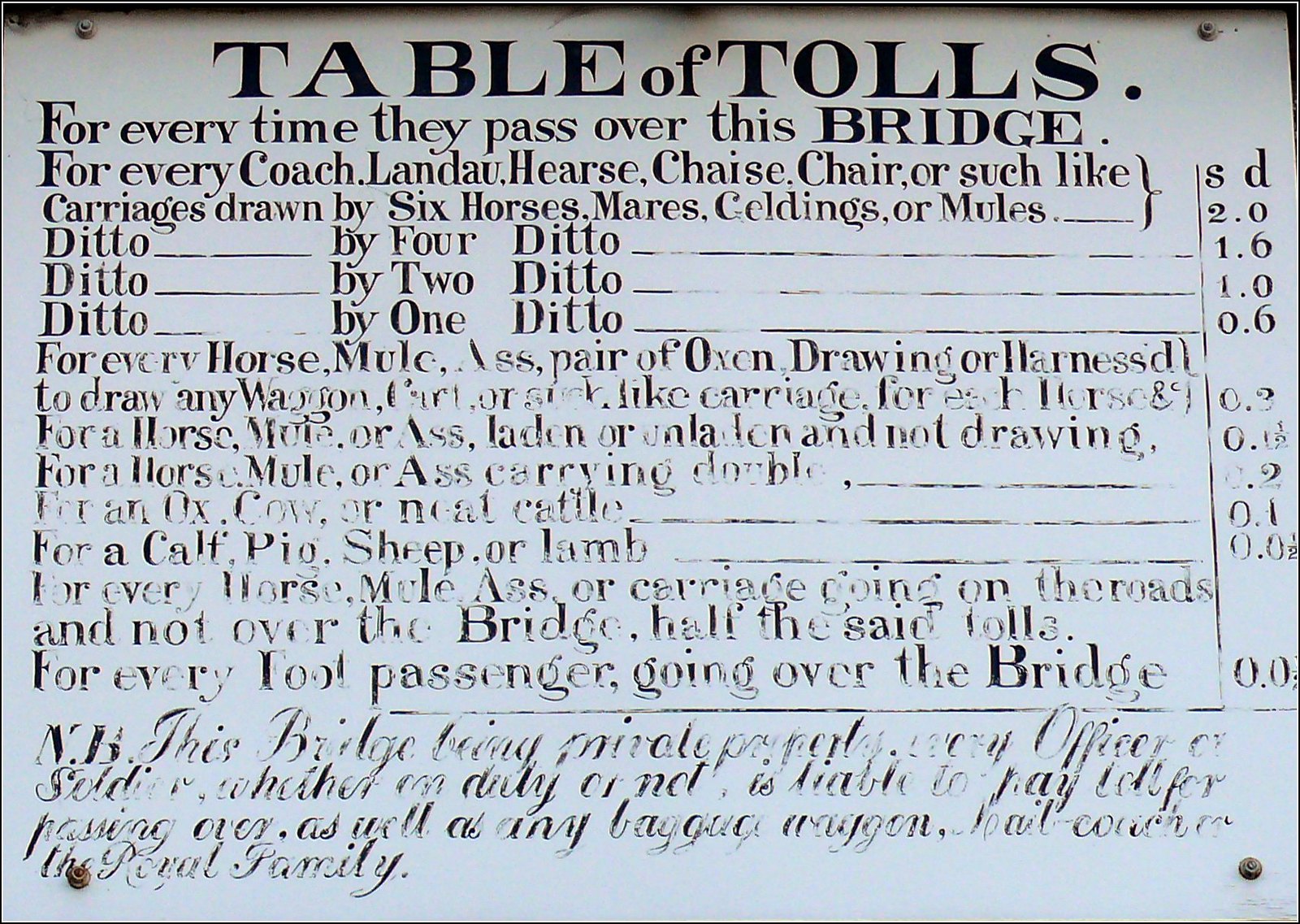This image showcases an old, weather-beaten metal sign advertising a toll bridge. The sign, off-white in color, is fastened with rusted metal bolts at each corner. A faint shadow runs across the top. In dark brown letters, it prominently displays "Table of Tolls." Below, it details the tolls for crossing the bridge, starting with, "For every time they pass over this bridge," and then listing various carriages such as "coach, landau, hearse, chaise, chair," drawn by different numbers of animals ranging from "six horses, mares, geldings, or mules" down to "ditto by four, ditto by two, ditto by one."

On the right side, corresponding prices like "SD 2.0, 1.6, 1.0, 0.6" align with charges for each type of carriage. Additional text details tolls for other animals and vehicles, although parts of this information are blurred due to weathering, making specifics difficult to discern. This includes lines about "every horse, mule, ass, pair of oxen drawing, or harnessed to draw any wagon, cart," and various conditions for "horse, mule, or ass laden."

At the very bottom, in faded cursive, it states the bridge’s private ownership, noting that, "every officer or soldier, whether on duty or not, is liable to pay toll for passing over, as well as any baggage wagon," and mentions the "Royal Family." Due to extensive weathering, much of this lower text is barely readable, adding to the sign's aged and historical appearance.